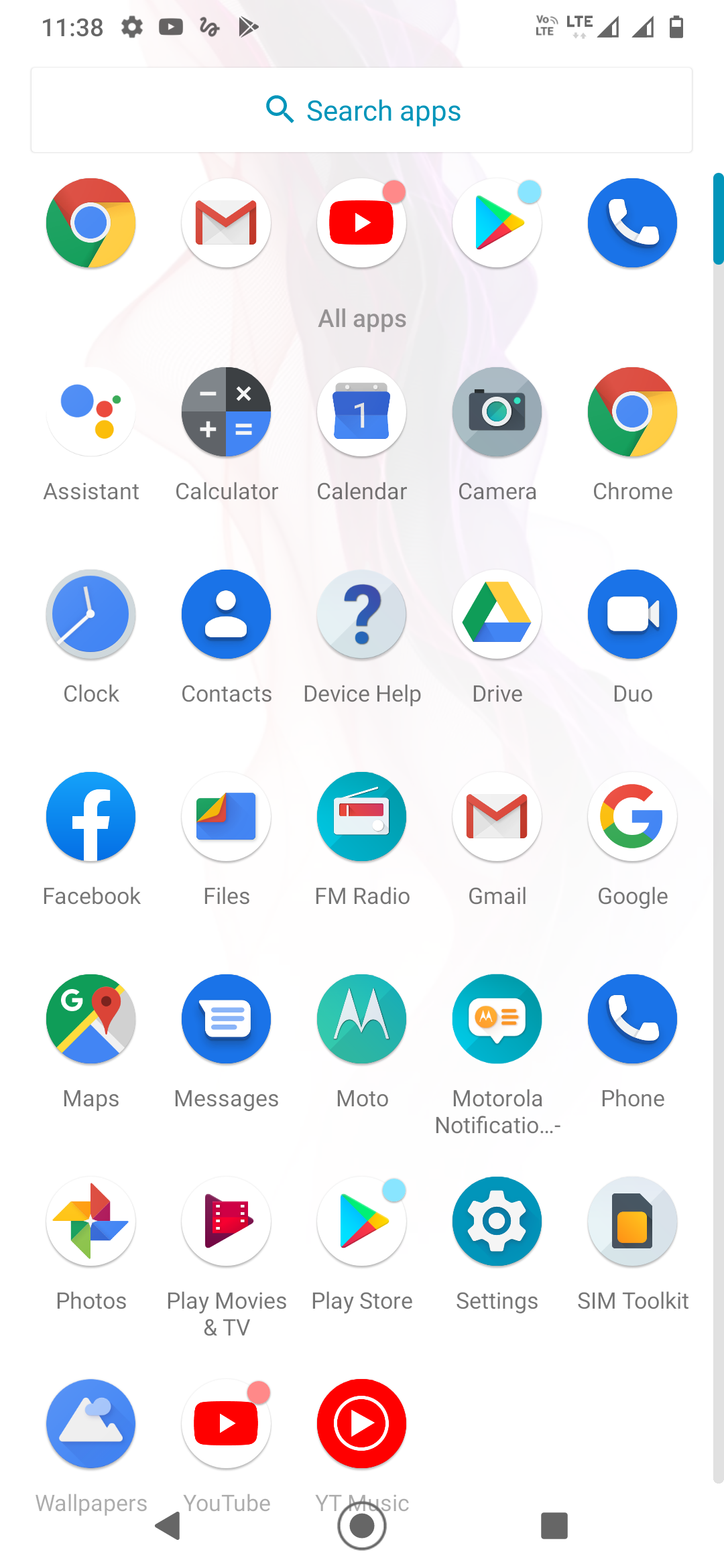Screenshot of a mobile phone home screen taken at 11:38 (time without AM/PM indicator). The phone is using LTE data with a visible signal strength indicator and battery level. At the top, there is a search bar labeled "Search apps" for easy navigation to apps. The homescreen displays a variety of app icons, including pre-installed ones like Google Chrome, Gmail, YouTube, Google Play Store, and phone call functionality. Below these are downloaded apps listed as Google Assistant, Calculator, Calendar, Camera, Chrome, Clock, Contacts, Device Help, Drive, Duo, Facebook, Files, FM Radio, Gmail, Google Maps, Messages, Moto, Motorola Notification, Phone, Photos, Play Movies & TV, Play Store, Settings, SIM Toolkit, Wallpapers, YouTube, and YouTube Music. The bottom navigation bar shows icons for 'Back,' 'Home,' and a square-shaped 'Recent Apps' button.